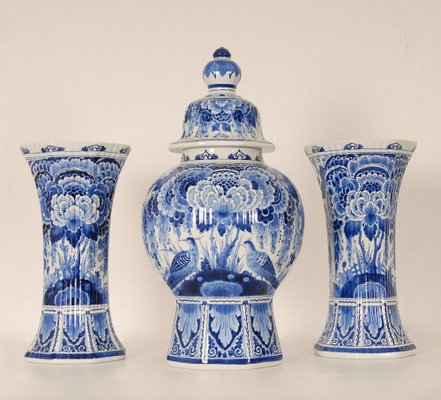The photograph showcases a set of three exquisite vintage Chinese porcelain pieces against a cream-colored background. Centrally positioned is a larger ginger jar with a rounded midsection and a decorative dome top. This jar features intricate designs depicting peacocks under stylized clouds and trees, complemented by a detailed pedestal base adorned with stylized acanthus leaves. Flanking the ginger jar are two identical vases, characterized by their columnar shape that slightly flares at both the foot and mouth. These vases are open at the top and exhibit similar blue and white floral and bird motifs, matching the central ginger jar's theme. The rims of all three pieces are aligned at the same height, showcasing a consistent white and blue pattern. These beautifully designed collectibles, likely bone china, are set on a flat surface and their delicate craftsmanship highlights their fragility and value to collectors.